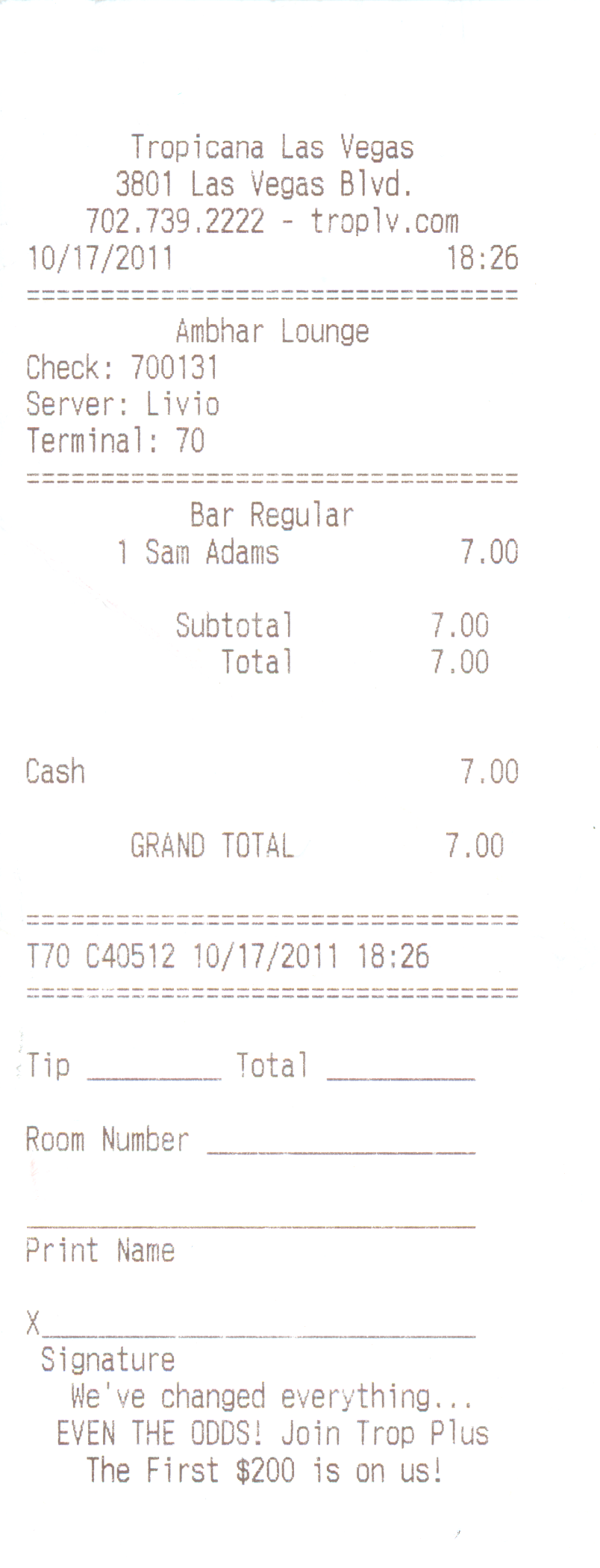This is a detailed picture of a receipt from the Ambar Lounge at Tropicana Las Vegas, located at 3801 Las Vegas Boulevard. The contact details include a phone number (702-739-2222) and a website (troplv.com). The transaction occurred on October 17, 2011, at 6:26 PM (18:26 in 24-hour time). The receipt shows a single purchase of a Samuel Adams beer for $7.00, which served as both the subtotal and the grand total. The payment was made in cash, and no tip was added. There is no room number, signature, or customer's name on the receipt. At the bottom, an advertisement reads, "We've changed everything, even the odds. Join Tropicana Plus. The first $200 in bets are on us." The receipt's white background blends into the surrounding environment, making its edges indistinct.